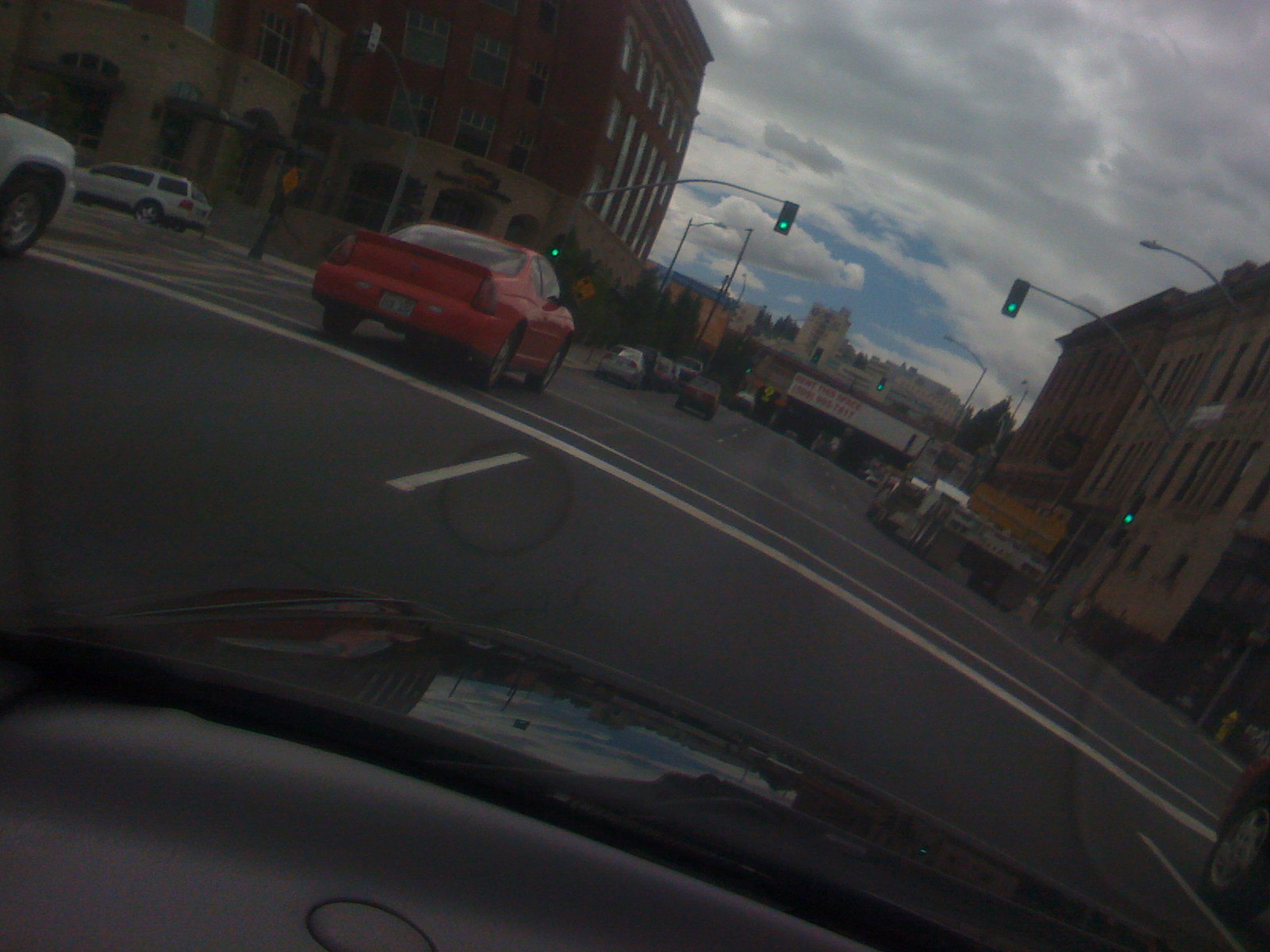In this detailed photograph taken from the driver's seat, likely through a dashboard camera or phone, we see an urban downtown setting on a clear yet somewhat hazy midday. The central focus is a green traffic light directly in front, with four signs indicating traffic may proceed. Immediately in front, a red compact sedan is crossing a marked crosswalk, while further down the one-way street cars are parked on the left and traveling ahead. Surrounding the street are older, double-story brick buildings on both sides, suggesting historical architecture possibly dating back 1,500 years. Notable among them is a white SUV parked to the left.

A marquee, possibly of a movie theater, stands prominent at a block's end, featuring illegible red lettering from this distance. To the right of the frame, partially visible, is a construction vehicle. Above, the sky is bright blue filled with clouds, adding a contrast to the slightly gloomy ambiance of the scene. The overall angle of the image feels slightly tilted to the left, adding to the dynamic and somewhat off-kilter composition of the photograph.